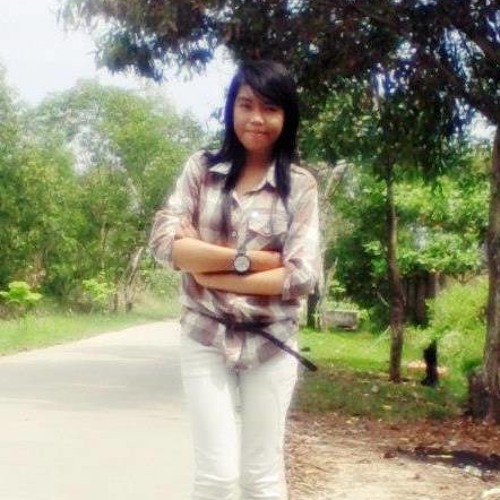A young Southeast Asian woman stands confidently on a narrow, light-colored paved path surrounded by dense woods and foliage. She has medium-length black hair with side-swept bangs that extend past her shoulders. Her face is round and she's smiling warmly at the camera. Dressed in a plaid flannel shirt with the sleeves rolled up to her elbows and unbuttoned at the very top, she cinches her waist with a thin black belt. She pairs the shirt with light-colored jeans and sports a large watch with a white face on her right wrist. Her arms are crossed in front of her as she stands amid trees and vegetation, with a clear walkway beneath her and a background of trees and a bluish-white sky. The right side of the path lacks vegetation, revealing dirt and dead leaves.